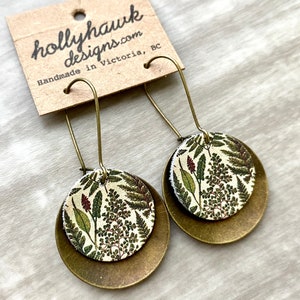This image is a detailed close-up of a pair of handmade, pierced earrings attached to a light brown cardboard tag. The tag is situated towards the upper left corner of the image and has a cut-off upper right corner. It features dark text that reads "hollyhockdesigns.com" in cursive, and "handmade in Victoria, BC" in a typewriter-like font. The cardboard also has a hole punched at the top center, presumably for hanging on a display peg.

The earrings themselves are made of gold metal and are designed to be looped into the ears. Each earring consists of two circles: a larger, reflective brass or bronze circle at the top and a slightly smaller circle below, decorated with intricate foliage prints. The foliage patterns are varied, featuring different types of leaves, including thick, thin, small, and fern-like leaves in green and brown tones. The surface on which the earrings and cardboard tag rest is a gray streaky wooden texture, adding a rustic element to the presentation.